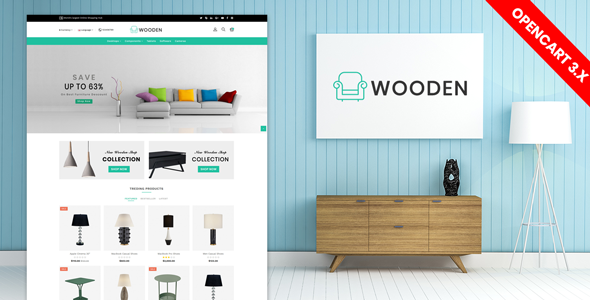This image is a detailed screenshot from a website called "Wooden." The background primarily showcases a room with vertical panels painted a light blue, giving the appearance of either woodwork or some type of siding. On the left-hand side of the screenshot, the website interface is overlaid. 

At the top of this web page is the name "Wooden" accompanied by an icon of a blue chair. Directly below this, the text "Save up to 63%" is prominently displayed. Moving further down, there's an image of a couch adorned with five colorful pillows in shades like purple, blue, and red.

The web page features several sections with slightly blurry text. Beneath the couch image, there are photos of two overhead lamps with the readable word "collection" associated with them. Next to these lamps, there's an image that most likely depicts a table with black legs.

In the following section, a series of lamp images are listed. They include a black-shaded lamp, a white-shaded lamp, another black-shaded lamp, and a fourth lamp with a white shade and black base. Below these, four additional lamp images are displayed.

On the right side of the page, there is a picture of an armchair next to the "Wooden" brand name again. Adjacent to the armchair, a small table is visible, supporting a black statue. Additionally, there is an upright lamp with a white shade and five metal legs, completing the scene.